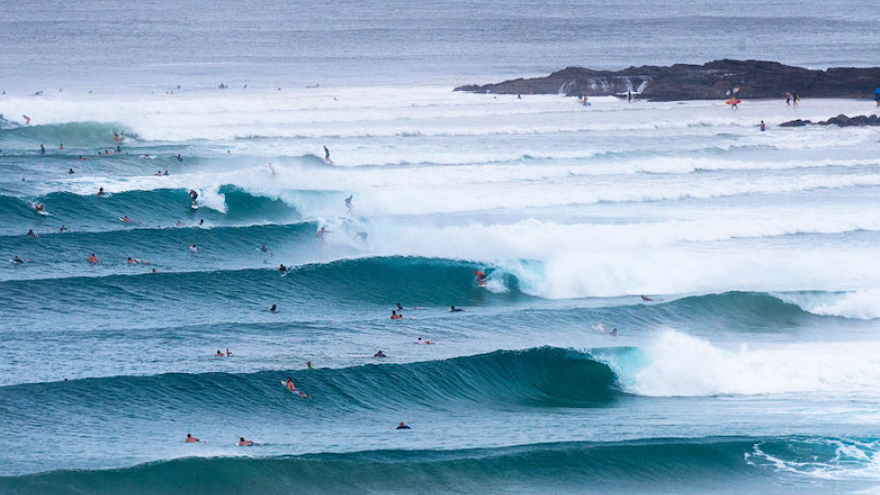The image captures a stunning seaside scene with a series of waves rolling towards a beach. In the foreground, the waves are just starting to wash up on the shore, creating frothy white water, while in the distance, a continuous flow of waves stretches as far as the eye can see. The left side of the image prominently displays thick, blue water where the waves are clearly visible, while the right side glows with bright sunlight, making the tops of the waves appear pure white.

In the far background, the horizon is distinguishable, separating the calm grayish-blue sky above from the expansive ocean below. In the upper right corner, there's a rocky projection or small island with jagged cliffs and possibly some people, who appear to be surfing or just standing near the edge. In front of this larger, mountainous landmass, a smaller ridge of rocks juts out into the water.

Scattered through the waves, various people can be seen surfing on their boards, floating in the water, or simply catching the next wave. Some of the surfers are just below the crests of waves that are breaking, adding dynamism and life to the scene. While the left side of the scene is more dominated by clear, darker blue water and defined waves, the right side transitions to frothy white water, especially near the bottom right corner where the water meets the beach.

Numerous people are depicted enjoying the ocean, with an estimated crowd of 50 to 100 individuals either surfing or swimming. The vantage point of the camera, likely taken from an elevated position or an aerial shot, beautifully showcases the energy and activity of this sunny daytime beach, capturing both the power of the ocean and the leisure of beachgoers.